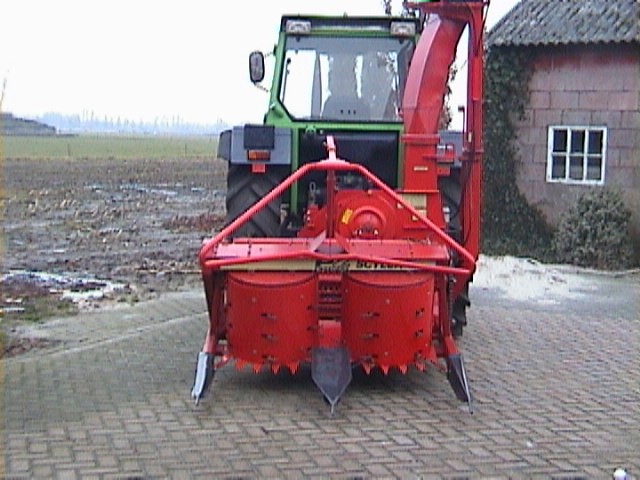The photograph features a piece of heavy machinery, specifically a green, enclosed tractor equipped with a red wood chipper attachment at the back. The tractor, complete with large wheels, roof, and glass windshields, is parked on a light tan, brick-paved surface. The wood chipper, identifiable by its red color and cylindrical components with spikes for chipping wood, also includes an adjustable angle chute for directing the wood chips. Dominating the background on the right is a bricked house with ivy and shrubs climbing its walls, and a corrugated metal roof with a single window that has six panes. On the left side of the background lies a muddy, barren field, possibly soaked from recently melted snow, adding a rough, open texture to the scene.